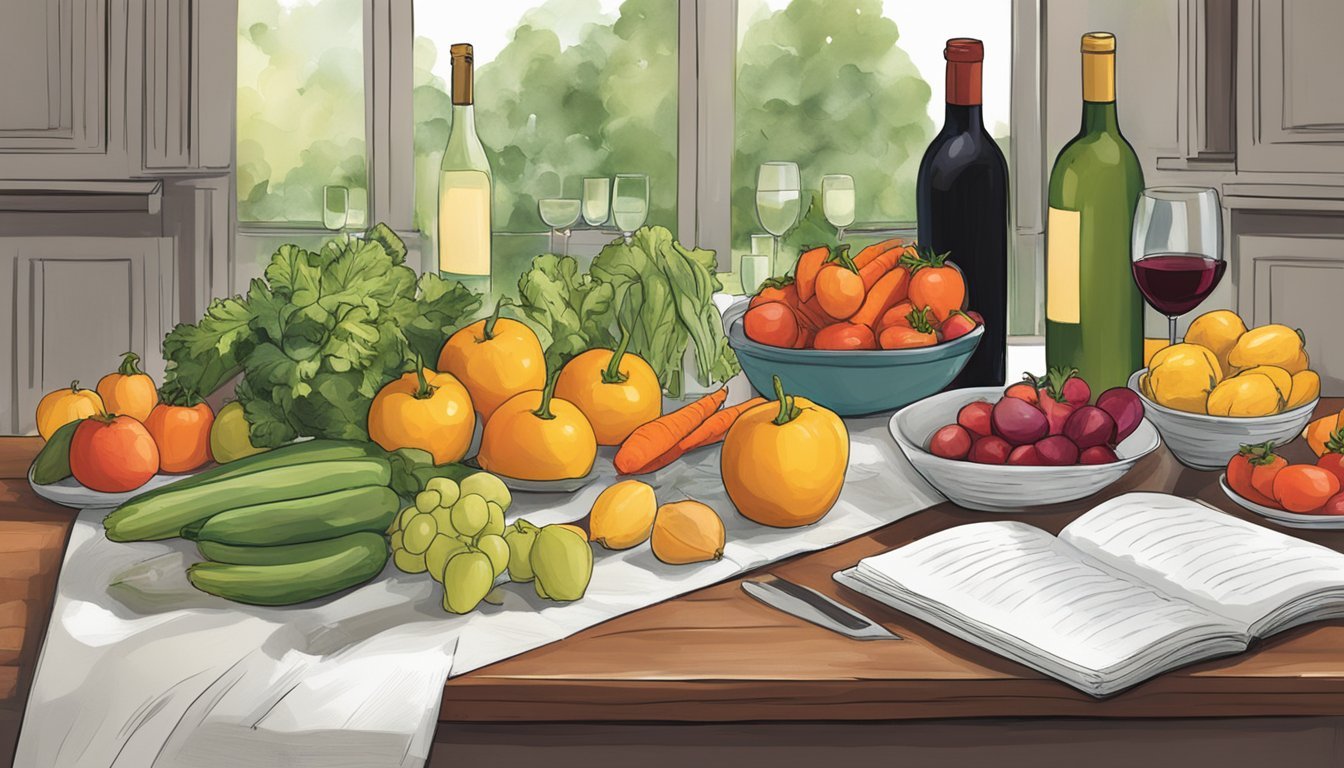This cartoonish illustration depicts a wooden dining table set in a daytime environment, likely a dining room with a view into a garden or an area with plants through a window. The background features a wall with some wooden fixtures and lush vegetation visible outside. The table is cluttered with various items, including an open book that may be a recipe book, fruits, and vegetables. Prominently displayed are tomatoes, cabbage, lettuce, and cucumbers. There are three wine bottles present—two appear to be red wine and one might be white wine. Additionally, there is a wine glass partially filled with red wine. Despite the somewhat disorganized arrangement, the scene exudes a vibrant and inviting atmosphere.